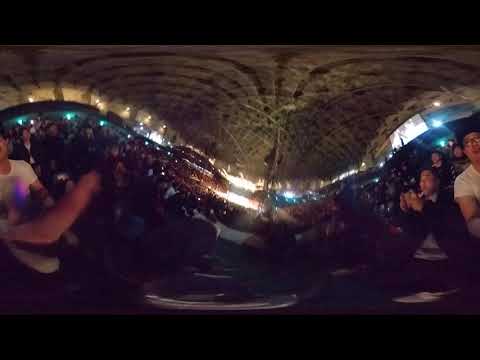The photo appears to be taken inside a dark, atmospheric venue resembling a club or concert hall. The room is filled with a large, indistinct crowd, suggesting a lively gathering possibly for a show or concert. The image suffers from blurriness and distortion, particularly notable in the background where people are harder to distinguish due to poor lighting and distance. The ceiling features a wavy, winged-like pattern with blue lights accentuating its curves, which adds to the warped aesthetic of the scene. In the foreground, on the left side, a person wearing a white shirt is visible next to another individual who seems to be lighting a cigarette. On the right, a similar figure in a white shirt can be seen, suggesting a 360-degree perspective that has been stitched together. Despite the overall low quality of the image, the middle section appears smushed while the sides curve upwards, enhancing the surreal ambience of the venue. The crowd, though blurry, appears engaged and possibly excited, indicating a dynamic, energetic event.